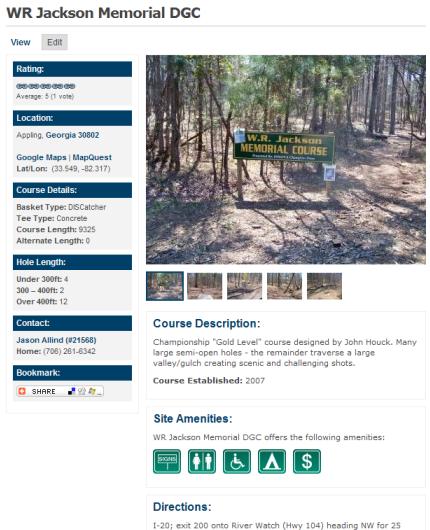This image captures detailed information about the W.R. Jackson Memorial Disc Golf Course located in Appling, Georgia, 30802. At the top, the page displays a "View" option and a gray "Edit" button. It provides a perfect average rating of 5 stars based on one vote. The geographic coordinates are given, and links to Google Maps and MapQuest are included for easy navigation.

Course details are meticulously listed with specifics such as basket type, Tee type listed as concrete, and a total course length of 9,325 feet. There is no alternate length. The hole lengths are categorized as follows: 4 holes are under 300 feet, 2 holes range from 300 to 400 feet, and 12 holes are over 400 feet.

The course is described as a championship gold-level course designed by John Houck, featuring a combination of large semi-open holes and challenging shots across a scenic large valley gulch. The course was established in 2007.

Additional site amenities include handicapped-accessible bathrooms, camping sites, and financial amenities, ensuring a comfortable experience for all visitors. Directions are provided at the bottom of the page for easy reference.

---

Detailed Descriptive Caption:
**A comprehensive overview of the W.R. Jackson Memorial Disc Golf Course in Appling, Georgia, showcasing its championship gold-level design by John Houck established in 2007. The course features large semi-open holes and challenging shots across a scenic valley gulch. It spans a length of 9,325 feet with hole ranges including 4 under 300 feet, 2 between 300 to 400 feet, and 12 exceeding 400 feet. The site includes valuable amenities such as handicapped-accessible bathrooms and camping sites, with detailed directions and mapping tools available for visitor convenience.**